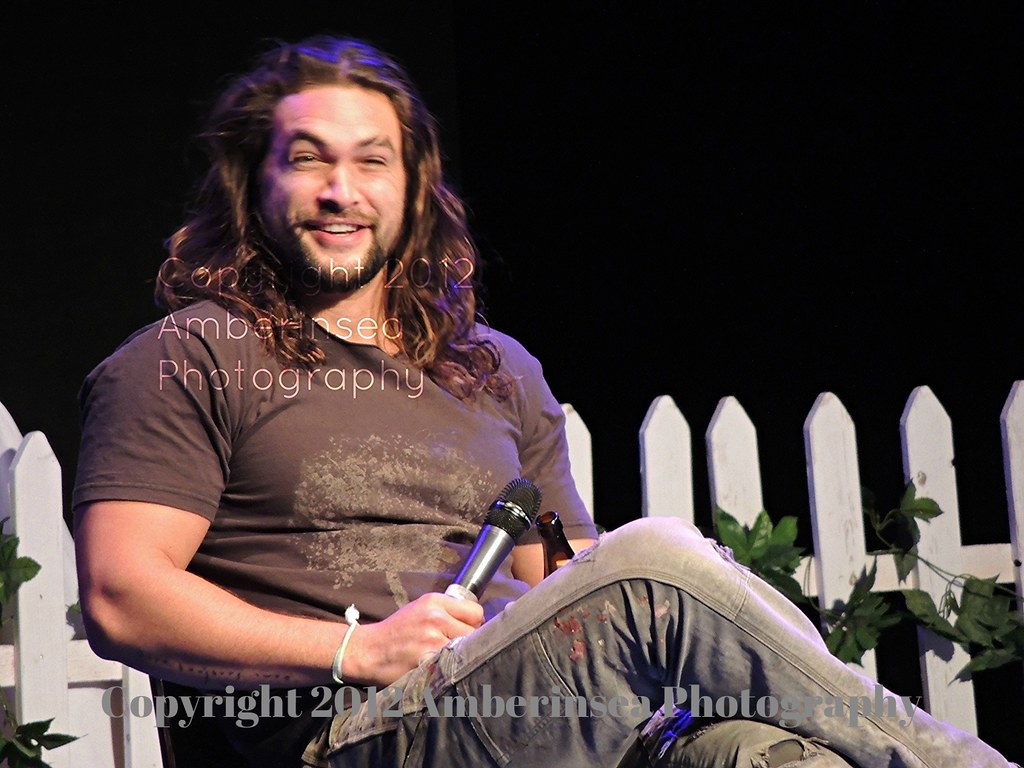This image captures Jason Momoa at a public event. He is seated with his right leg casually crossed over his left, holding a black microphone with a matching black top in his right hand, though not raised to his mouth. On his right wrist, he sports a white bracelet. Jason is dressed in a short-sleeved brown t-shirt adorned with a pattern resembling yellowish tree splotches. His distinctive facial hair frames his face, featuring a goatee or beard. His long hair cascades down to his shoulders, with the ends forming subtle curls.

He wears a pair of jeans that appear well-worn and covered in paint splatters, hinting at a creative or hands-on project, and they also feature slight rips. In his left hand, he holds a dark brown glass bottle, partially obscured by his bent leg. A focused light illuminates Jason, who is smiling or laughing warmly, though his gaze is directed past the camera, suggesting he is interacting with someone off-screen.

The backdrop is a striking black, complemented by a white picket fence adorned with artificial green foliage entwined around each picket. This detail, along with his relaxed demeanor, adds a touch of casual charm to the setting. The overall composition of the photo reflects a moment of candid engagement at the event.